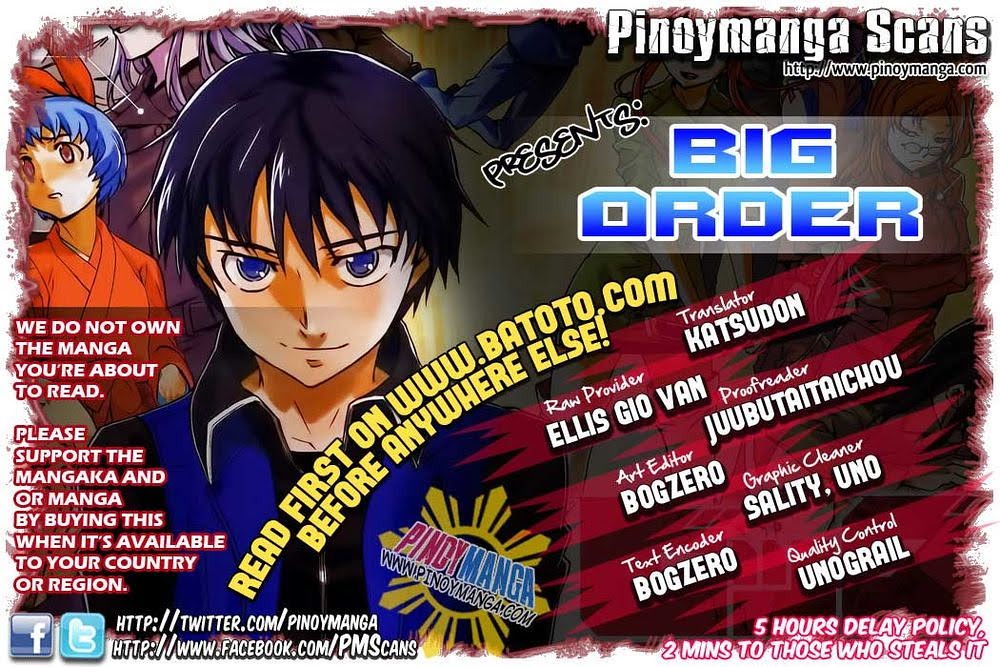This image is an advertisement for Pinoy Manga Scans, featuring prominently an anime-style graphic with multiple characters and extensive text detailing various credits. The background comprises red and gray banners. The central character, depicted from the chest up, captures immediate attention with their blue jacket, black collar, black shirt, dark gray hair, and striking blue eyes that gaze downward, seemingly making eye contact with the viewer. To the right (or left) is another character adorned in an orange robe with blue hair, looking off to the right.

In the upper right corner, white text against a blue background announces "Pinoyemanga Scans Presents Big Order." Below this title, on a red background with white text, are numerous credits including, "Translator: Kat Sudon, Raw Provider: Alice Gayo Van, Proofreader: Jubutai Taichu, Art Editor: BogZero, Graphic Cleaner: Sality Uno, Text Encoder: BogZero, Quality Control: UnoGrail." The left side of the image contains a message urging support for the mangaka by purchasing the manga when available and providing additional details on reading the content first on www.batoto.com. Facebook and Twitter logos with corresponding URLs are displayed at the bottom, promoting the social media presence of Pinoy Manga Scans. Additionally, the lower right corner features a note about a "Five Hours Delay Policy" and a brief warning regarding content theft.